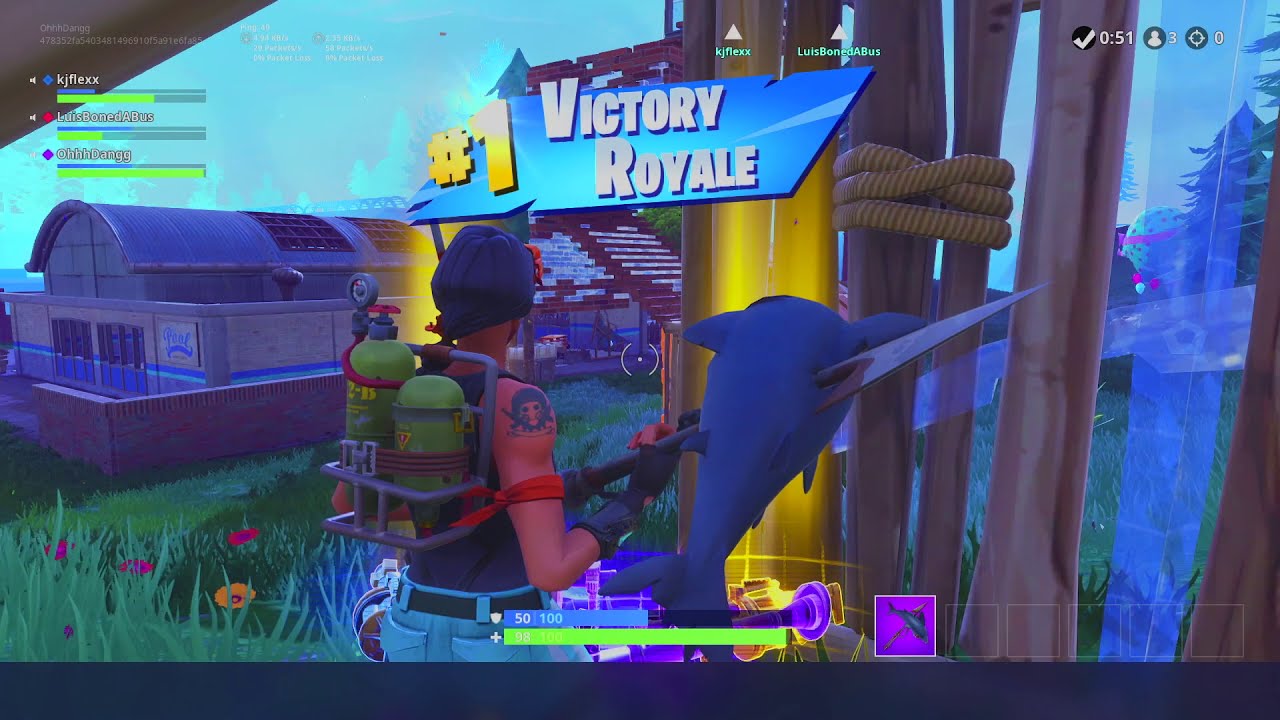This detailed screenshot from the video game Fortnite displays a vibrant, digital battleground. The wide rectangular image is partially cropped at the bottom by a dark blue strip, focusing attention on the dynamic scene. Dominating the background, a vivid green lawn stretches under a bright blue sky, with multiple buildings encircling the area. 

On the left side, a distinctive greyish-brown domed building stands, enclosed by a wooden fence with grey accents, fronted by a short red and grey brick wall featuring entry points. To the right, several tall wooden planks, some fastened by light yellow wood, create a rustic contrast.

At the center, a female character with a ponytail and tattoos stands facing away from the camera. She is equipped with a black hat and carries a set of green air tanks encased in metal on her back. She wields a long spear, skewering a blue creature at the tip. Above her head, the text "Victory Royale number 1" is boldly displayed in white and yellow on a blue background, signifying a triumphant moment.

Additional text at the top includes "KJ flex Lewis boned a bus" and "oh dang," contributing to the layered visual storytelling. The array of colors, including blue, green, red, yellow, grey, and brown, enriches the overall digital artwork, reinforcing the game's dynamic and animated style.